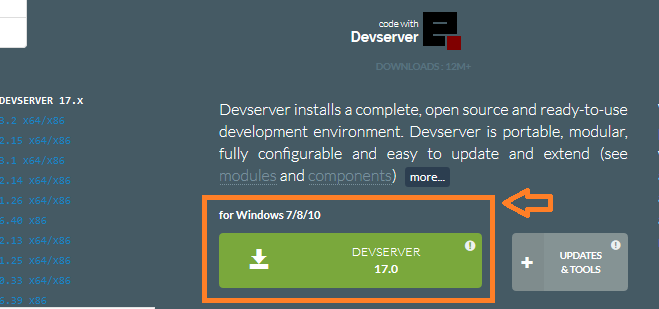This image displays a heavily cropped section from a website, featuring what appears to be a page dedicated to updates or downloads for a software tool named "Deserver." The background is gray, and the left side of the image showcases different build versions of the software, with clickable blue links. At the top of the image, the text reads "Code with Deserver," accompanied by a black and red logo to the right. Below this, there is a statement indicating that the software has "12 million downloads." 

A detailed description of Deserver follows: "Deserver installs a complete open source and ready-to-use development environment. Deserver is portable, modular, fully configurable, and easy to update and extend. See modules and components." Underneath this, an orange box highlights the text "For Windows 7, 8, and 10" alongside "Deserver 17.0." This section also features a large download button on the left, and to the right, there are buttons labeled "Update" and "Tools." An orange arrow points directly to the prominent download button, drawing attention to it.